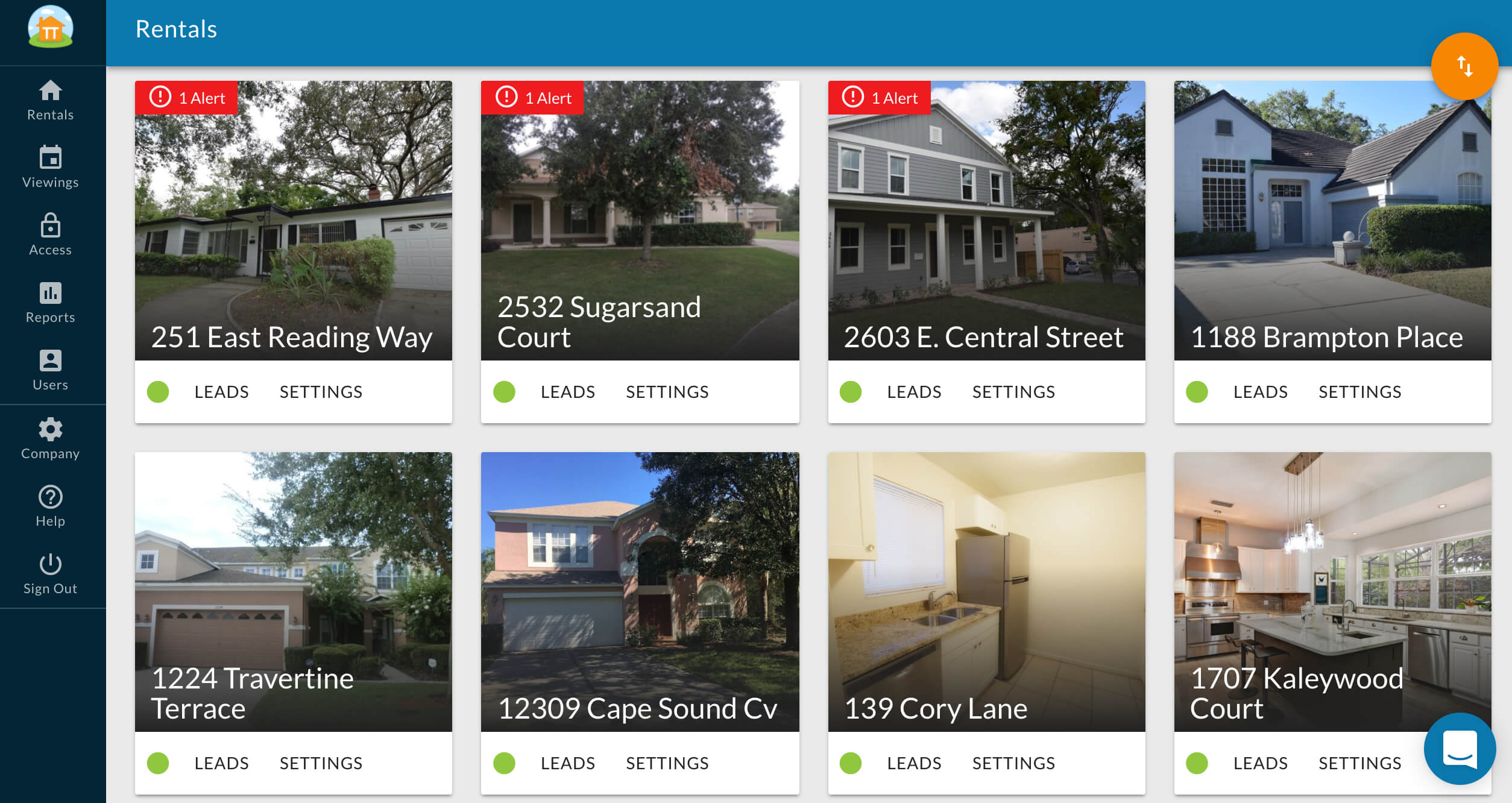The image showcases a website dedicated to aggregating rental property information from various sources. The layout features a dark blue vertical rectangle on the left-hand side, prominently displaying a small circular logo at the top. The logo depicts an illustrated house in orange, accompanied by green grass and a blue sky. To the right of this vertical bar, a royal blue horizontal rectangle spans the page's width, excluding the section adjacent to the dark blue bar. Within this blue band, the word "Rentals" is prominently displayed in a crisp white font. Below this header, eight thumbnail images of available rental houses populate the main section, representing properties in the searched area (specific location not indicated). Notably, three of these thumbnails have small red boxes in their upper left-hand corners, signaling recent activity or updates related to those particular listings.